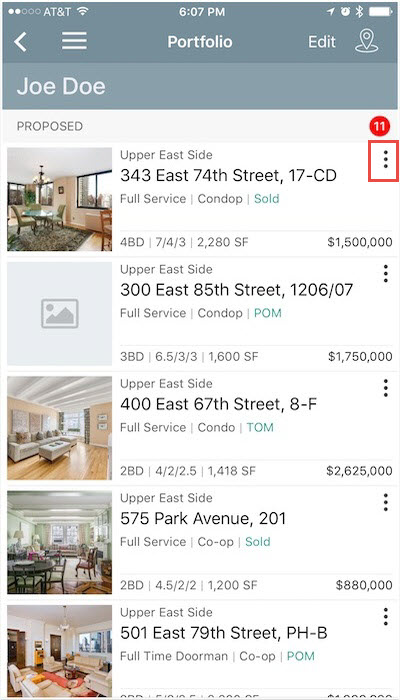The image depicts a smartphone screen displaying various real estate listings. The status bar at the top of the screen shows the time as 6:07 PM, with AT&T as the network provider, alongside icons for WiFi, Bluetooth, and battery percentage. Below the status bar, there are several navigational elements including a white back arrow, a button with three horizontal lines, a portfolio section, an edit button, and a location symbol. The heading on the screen reads "Jodo."

Under a section labeled "Proposed," the number 11 is displayed, indicating the number of listings. The listings are detailed as follows:

1. **Upper East Side, 343 East 74th Street, 17 CD**
   - Type: Full-service condop
   - Status: Sold
   - Size: 2,280 square feet
   - Price: $1.5 million

2. **Upper East Side, 300 East 85th Street**
   - Type: Full-service condop
   - Size: 1,600 square feet
   - Price: $1.75 million
   - Status: Sold

3. **400 East 67th Street, 28D**
   - Type: Full-service condo
   - Size: 1,418 square feet
   - Price: $2,625,000

4. **575 Park Avenue**
   - Size: 1,200 square feet
   - Price: $880,000
   - Status: Sold

5. **501 East 79th Street**
   - Type: Full-time doorman
   - A thumbnail image shows a living space with a couch, windows, and hardwood flooring.

The majority of the page has a clean, white background, providing a clear view of the listings and details.